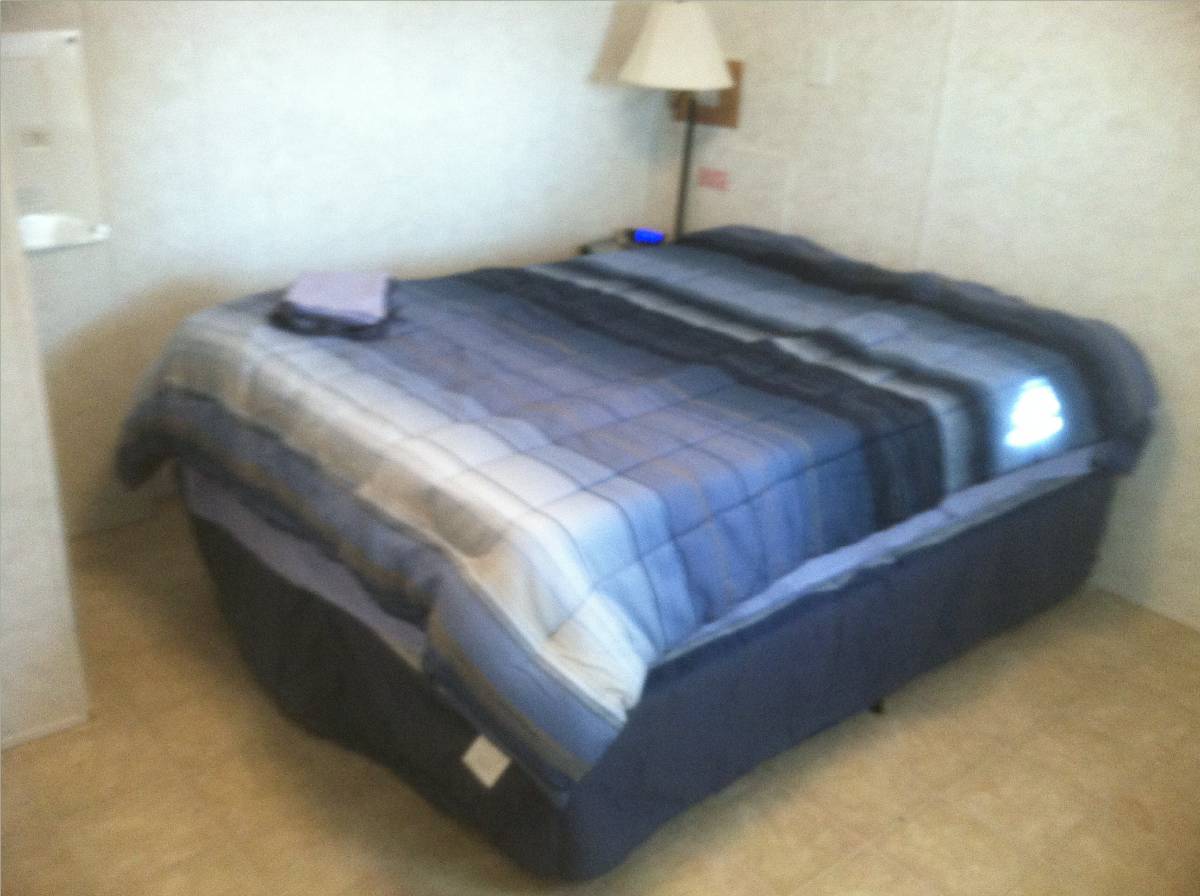This somewhat out-of-focus photograph depicts a small motel room with a full-size bed. The plain beige walls and brown rug define the simple decor. The bed comprises a dark blue box spring and a mattress covered with a blue, black, and white striped duvet, although it's somewhat wrinkled and not crisply made. At the foot of the bed lie two folded towels, one pink and one dark blue. A small bedside table stands adjacent to the bed, holding an electronic display clock and a lamp. The floor seems to be covered with yellow tiles, adding to the room's modest and understated aesthetic. No pillows are on the bed, and a section of the wall or an opened door is faintly visible on the left.